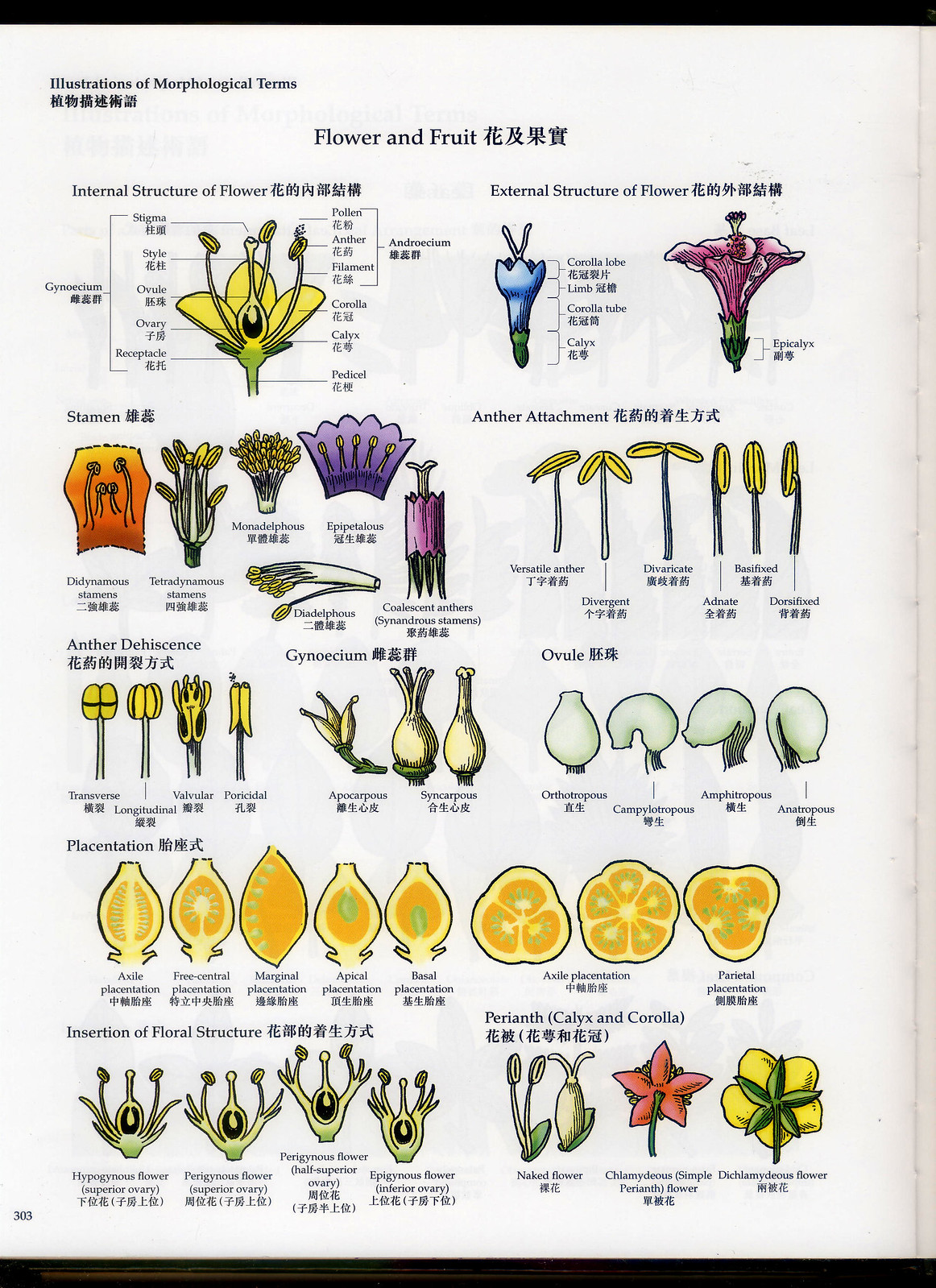This image appears to be a detailed page from a book, likely a botanical textbook with some Chinese text. Titled "Illustrations of Morphological Terms" at the upper left corner and "Flower and Fruit" across the top, the page features numerous labeled diagrams of flowers, fruits, and vegetables. These are not actual photos but seem to be pencil drawings filled with various colors such as yellow, orange, blue, purple, pink, and green. The page meticulously breaks down and labels the internal and external structures of flowers, including specific parts like stamina and the attachment points. Additionally, it covers the growth cycle and various aspects of these plants, illustrated with around 11 to 12 distinct diagrams, making it a colorful and comprehensive study tool.